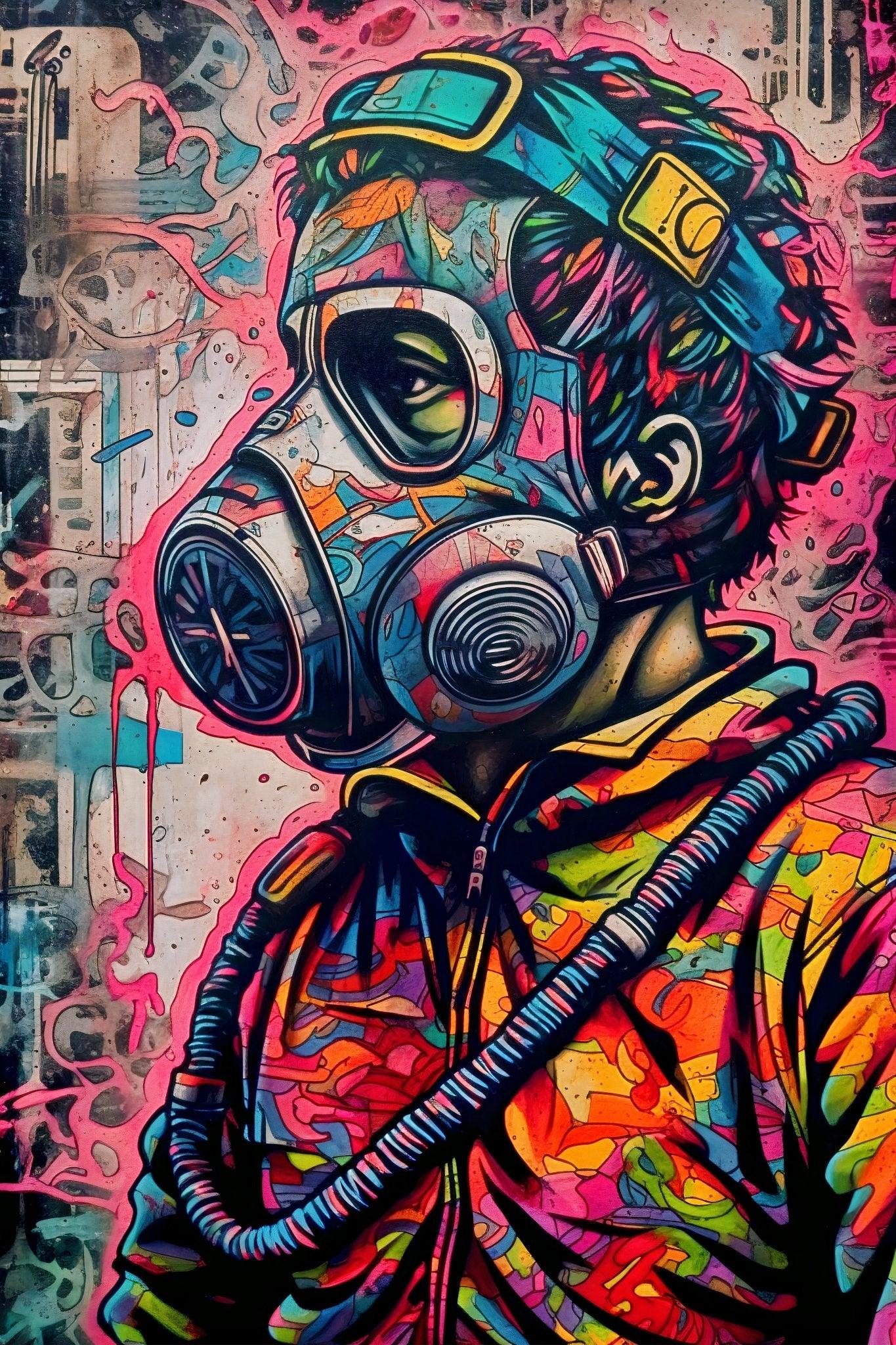This vibrant and detailed artwork features a human male in profile, his head turned to the left and his upper body slightly angled to display his colorful, zipped-up jacket, which exhibits a kaleidoscope of colors including yellows, oranges, reds, pinks, blues, greens, purples, and blacks. He is adorned with a necklace resembling candy beads from childhood, predominantly in blues and reds. Covering his face is a multicolored gas mask, with straps running around the back and lower head, and a hose extending over both shoulders. The background of the painting is an abstract array of splotches in pinks, blues, whites, grays, and off-white, enhancing the vibrant, expressive nature of the piece. The artwork, lacking any text or words, presents a richly colorful vision that captivates and evokes a sense of imaginative, artistic expression.